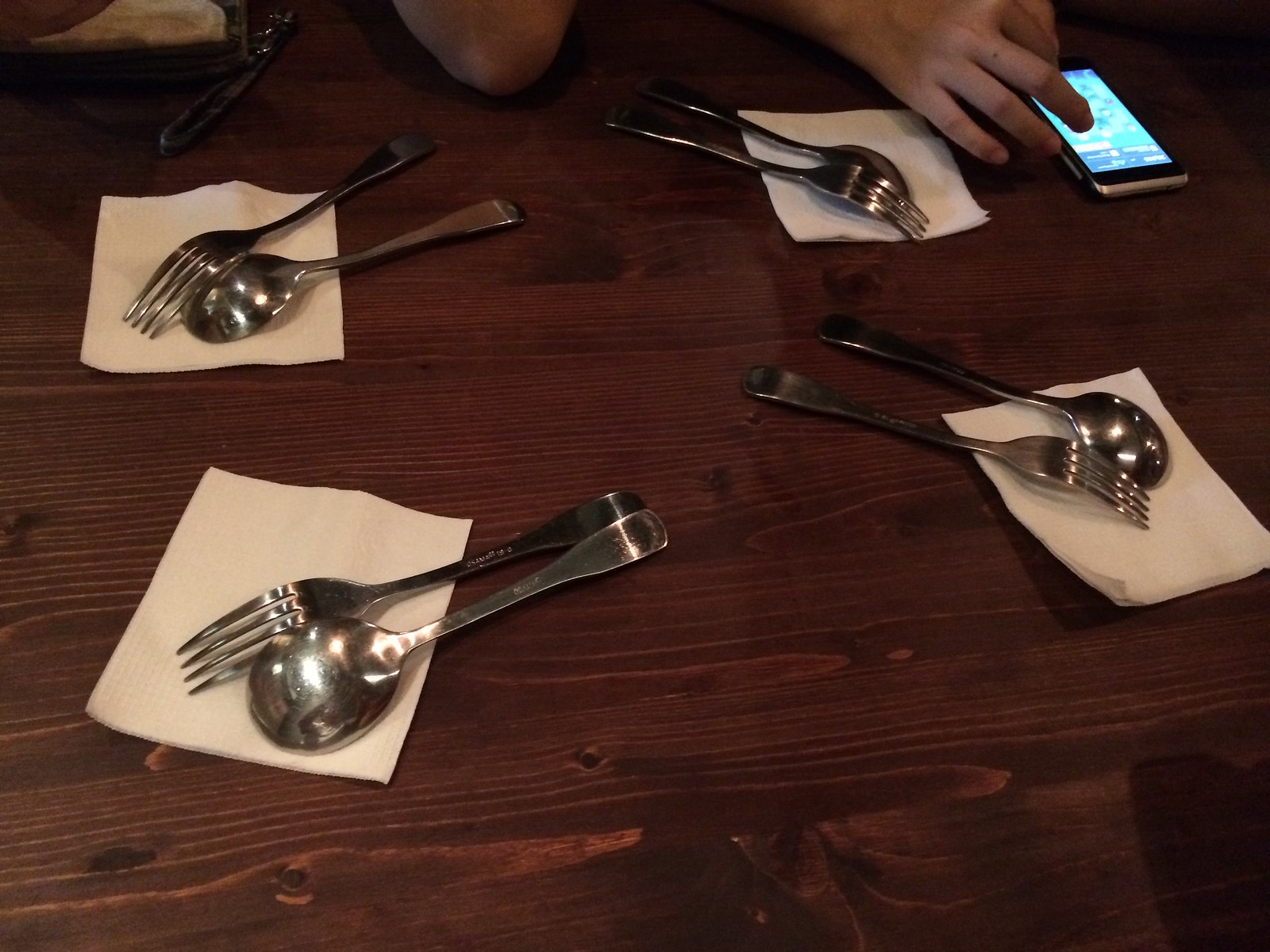The image features a dark wooden, picnic-style table adorned with four small beverage napkins placed near the corners. Each napkin pairs a metal fork and a soup spoon, with the utensils facing downwards—the prongs of the forks and the bowls of the spoons are touching the napkins. Two pairs are positioned diagonally in one direction, while the other two are angled differently. In the upper right corner, a hand with a finger hovering over a lit touchscreen smartphone suggests the person might be scrolling. Near the center-right, a tan elbow rests on the table, likely belonging to the individual using the phone, though another elbow is also visible, implying the presence of another person. In the upper left corner, there is a white object resembling a wallet with a strap, contributing to the casual and laid-back scene.